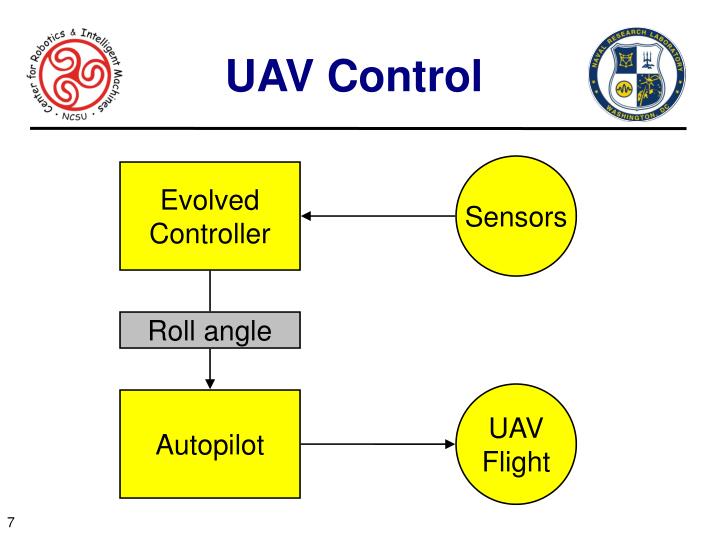The image depicts a structured presentation slide designed for a technical audience, likely part of a PowerPoint presentation. The main title "UAV Control" is prominently displayed at the top in blue capital letters. Flanking this title, there are two circular logos: the left logo is red and features the text "Center for Robotics and Intelligent Machines, NCSU" curving around its border, while the right logo displays the text "Naval Research Laboratory, Washington, D.C." in yellow letters on a blue background featuring a shield design with additional yellow symbols.

Below the title, a horizontal black line stretches across the slide, delineating the header from the main content. The content below is an organized flow chart with interconnected shapes, suggesting a control system schematic. On the left, three vertically aligned rectangles are sequentially labeled: "Evolved Controller" in black text on a yellow background, "Roll Angle" in black text on a gray background, and "Autopilot" in black text on a yellow background. The sequence continues with an arrow pointing right to a circle labeled "UAV Flight" against a yellow background. An additional yellow circular shape labeled "Sensors" resides in the upper right corner, connected by an arrow pointing towards the "Evolved Controller" box, completing the logical flow of this control system diagram.